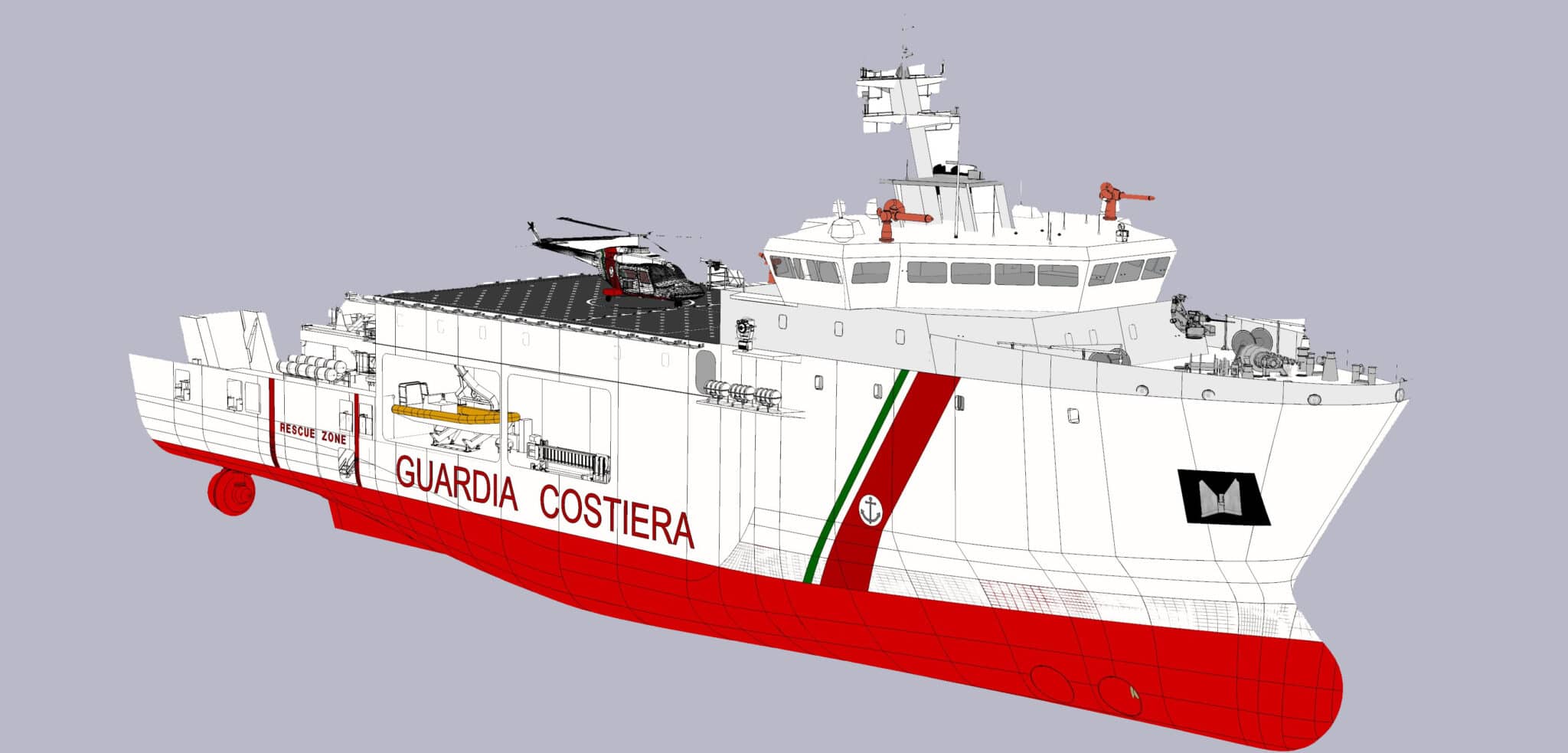This multicolor digital artwork features a detailed, horizontal, borderless depiction of a non-American Coast Guard vessel set against a gray background. The ship, primarily white with a red bottom, prominently displays the words "Guardia Costiera" in red along its side. A white, red, and green striped emblem adorned with an anchor symbol further accentuates the vessel’s bow. At the very bottom of the hull, the red coloring stands out. The ship’s superstructure is white, housing numerous windows at the top where the captain and crew would be situated. Several gun ports and possible water cannons are visible, adding a sense of readiness for engagement. Toward the stern, a black helipad supports a black helicopter, while the term "Rescue Zone" is marked in red at the back. The absence of water emphasizes that the drawing or painting is a precise representation of the ship out of water, capturing all intricate details such as the propeller at the very rear and various features that would be essential in a real-life maritime rescue scenario.